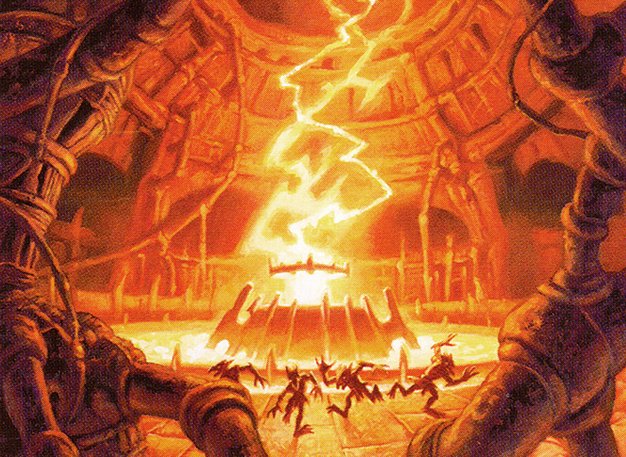In this detailed, fiery, and fantastical scene, the image portrays a hellish lair or dome-like interior, reminiscent of both sci-fi and fantasy worlds. The overall color scheme is dominated by intense oranges, reds, and yellows, evoking the sense of a place engulfed by hellfire. At the heart of this infernal environment stands a large altar or mechanism, with a striking lightning bolt emanating straight upwards from the center, hitting a pool of molten lava or molten metal.

The structure itself seems to be a disrepair-ridden mix of stone and discarded machinery, with metal ducts and pipes extending from the walls, contributing to its ominous atmosphere. This entire chamber appears fiery and chaotic, with a high level of heat and energy.

Running around or away from the altar are small, demon-like creatures, with features that could be interpreted as large ears, horns, or even bat-like appearances, complete with arms and legs. Their frantic motion adds to the pandemonium of the scene. The chaotic setting gives the impression of a cross between a depiction of hell and a high-stakes sci-fi scenario, as if the environment is on the brink of some catastrophic event.